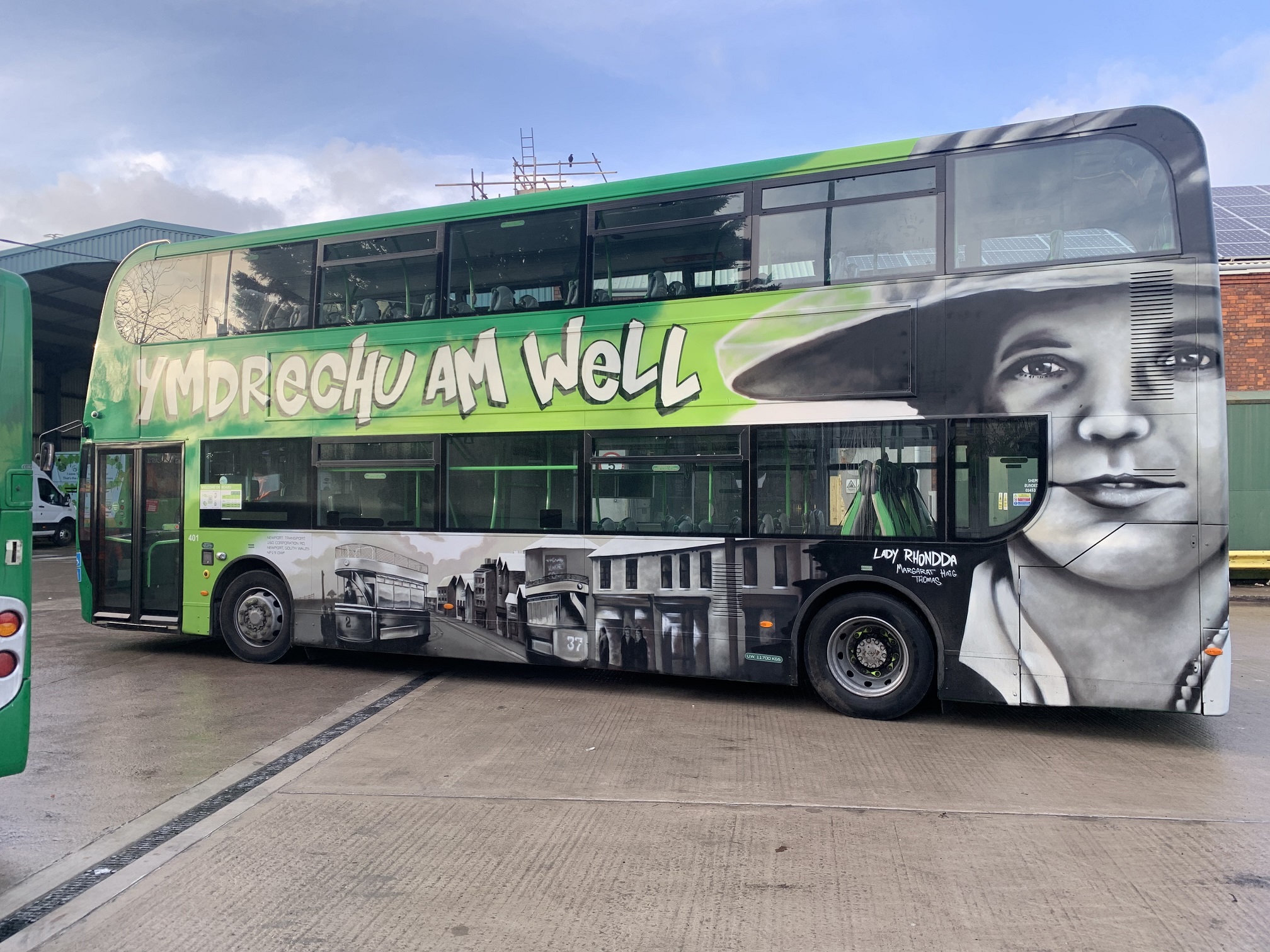The image depicts a bright grass green and deeper darker green double-decker bus with extensive advertising on its side. The bus features large white letters outlined in black spelling "YMDRECHU," with "AMWELL" following afterward. A distinctive black and white photo is integrated into the lower section and rear of the bus. This photo showcases a wide-brimmed hat-wearing young man with a slight smirk and a possible shell necklace, occupying a significant area in the back. Below this, the imagery transitions into a vintage street scene likely set in a Latin American country, depicting an antique double-decker bus and old-style buildings from the late 1800s or early 1900s. The bus also has large glass windows spanning both the upper and lower levels. The front area has double doors and a green strip separating the top and bottom windows. The bus is situated in a large concrete parking lot, with an adjacent partly brick and metal building featuring solar panels on the roof. Nearby sits another bus under an overhang designed for parked buses. The scene is set against a cloudy daytime sky with some scaffolding visible behind the bus.